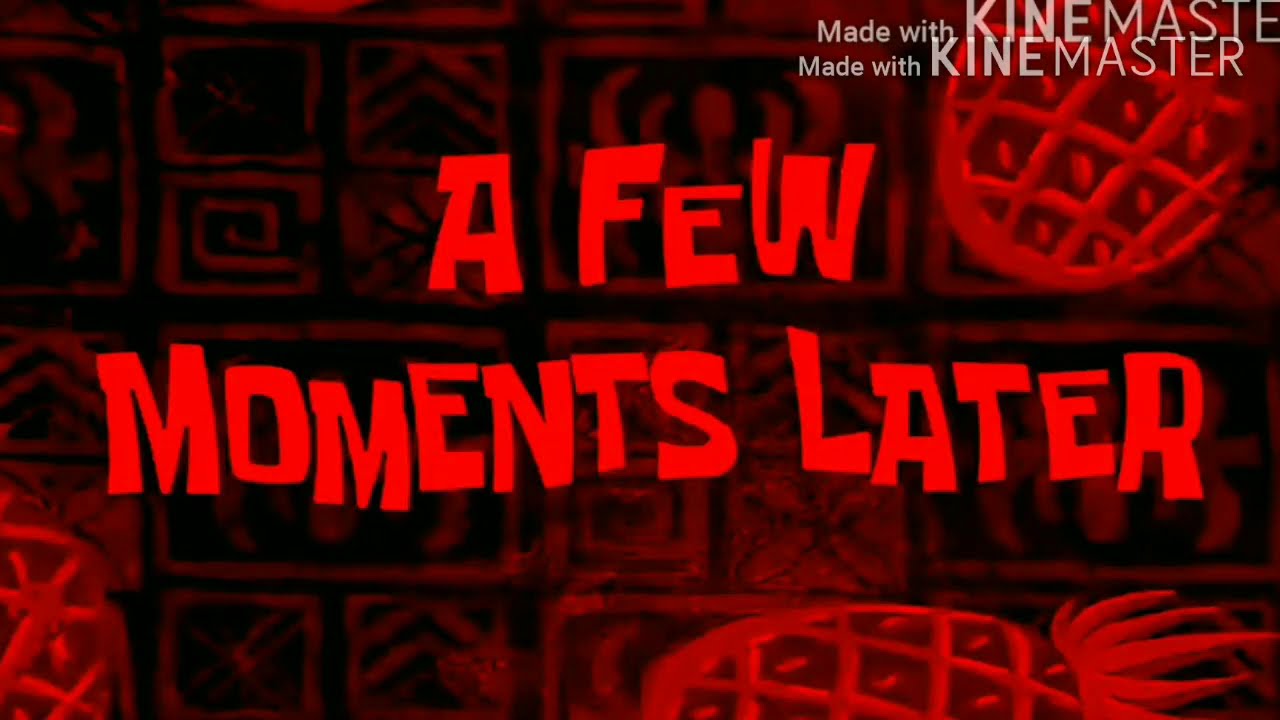The image is a cartoon-like drawing taken from a cut scene in the SpongeBob SquarePants television show. It features a predominantly red-tinted background with varying shades of red, creating a visually striking effect. The background consists of intricately designed tiles that resemble stone, many adorned with beautiful, albeit indistinguishable, patterns. Among these tiles are light red pineapples; one in the upper right-hand corner is plump with its top obscured, while another on the left lies on its side, clearly showing its top. Central to the image, in playful, youthful block letters commonly associated with SpongeBob SquarePants, is the text "A Few Moments Later." Additionally, the top right corner displays the white text "Made with KineMaster," a watermark that appears partially cut off. This still captures a classic meme-worthy moment from the show, now altered with an all-red tint as a creative twist.